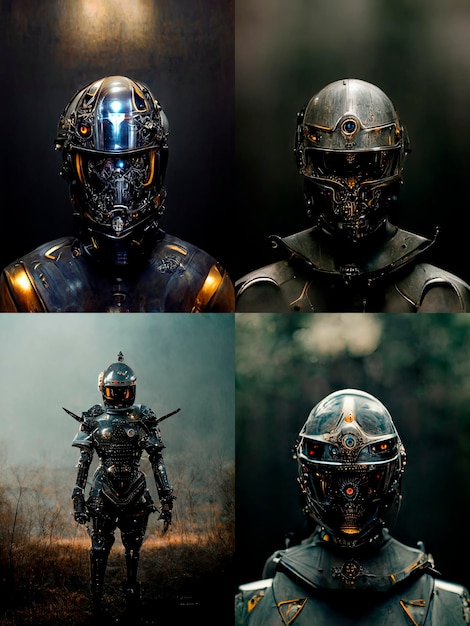This image is a collage of four distinct segments, each featuring a humanoid robot fighter in elaborate armor. The upper left segment showcases a robot fighter with a mean, stern appearance, adorned in metallic armor with blue, black, and gold hues, particularly around the shoulders and face, set against a dark gray background. In the adjacent upper right segment, another similar robot fighter is depicted with a muted steel-gray outfit and an abstract armor piece around the neck. A prominent blue circle adorns the center of the helmet, obscuring much of the face. Moving to the lower right, there is a robot fighter with bluish armor and a more decorated helmet featuring accents of red, yellow, orange, and green, giving it a gem-studded appearance. The blurred background adds to the mysterious ambiance. Lastly, the lower left quadrant presents a full-figured robot fighter, standing tall with swords on his back. He is clad in full armor, with distinctive spiky points on his shoulders, all set against a fiery prairie backdrop, hinting at a dramatic battle scene. The collage artfully combines these detailed robot fighters, each unique yet thematically cohesive in their metallic, combative designs.